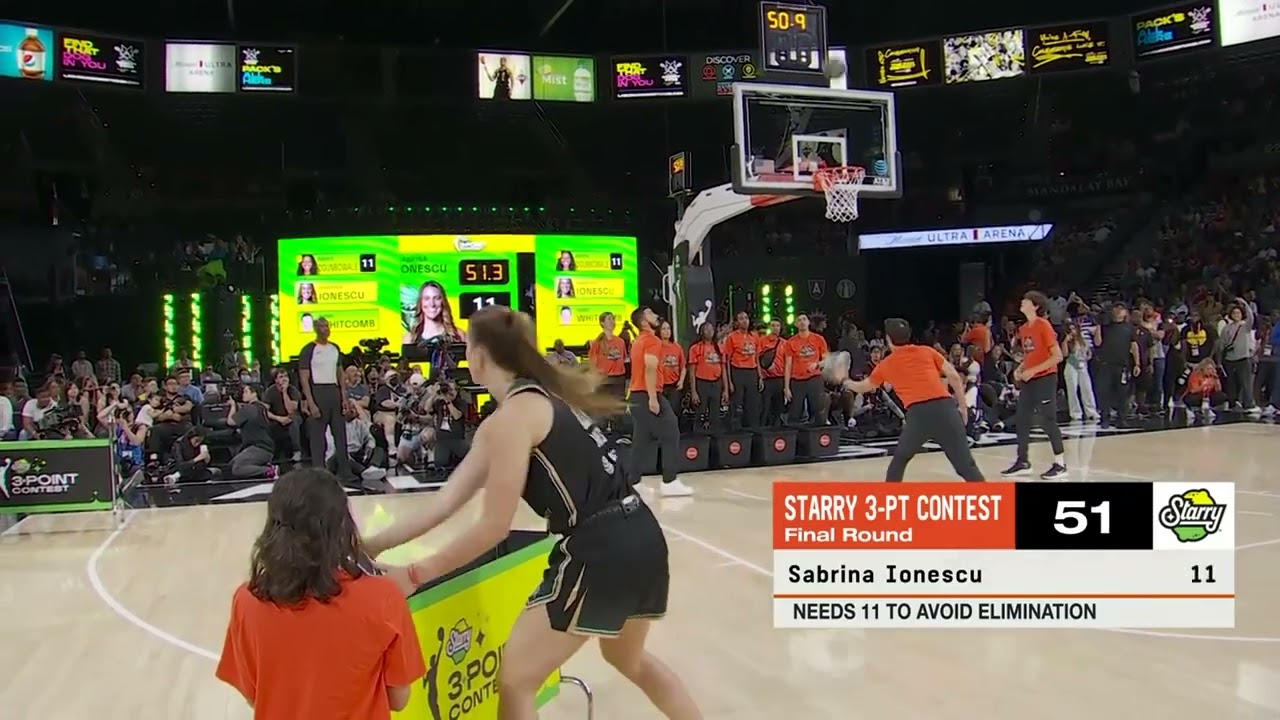The image captures a crucial moment at the WNBA All-Star game during the Starry Three-Point Contest final round. The focal point is Sabrina Ionescu, who is positioned on the court in a black jersey, preparing to make her next throw. She needs 11 points to avoid elimination and her current score is displayed as 51 points on the screen. Next to her, another player in an orange jersey stands near a table marked for the three-point contest. The scene is surrounded by a bustling arena, with men and women in orange T-shirts gathered closely under and around the basketball hoop, presumably to assist with rebounding the ball. Behind them, a packed audience watches attentively in the dimly lit venue. The arena is adorned with various vibrant advertisements and billboards, including a prominent green and yellow one displaying photos and stats of the players, all contributing to the electric atmosphere of the event. The scoreboard and the time clock above the backboard are also visible, adding to the detailed setup of this high-stakes competition.